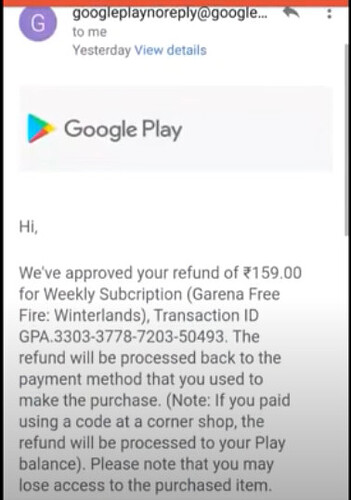Screenshot of an Email from Google Play Detailing Refund Approval:

At the top of the screenshot, a thin red bar is displayed horizontally across the screen. Below this, the email header shows "Google Play" represented by a purple circle with a white "G" on the left. The sender's address, "no-reply@google.com," is visible under the header, along with the recipient labeled as "me," the date marked as "yesterday," and a "View details" link in blue text beside it.

The main content of the email is in a light gray rectangular area. On the left side of this section, the Google Play logo - a triangle with the colors blue, red, yellow, and green - is prominently visible. 

The text within the email reads as follows: "Hi, we've approved your refund of ₹159.00 for Weekly Subscription (Garena Free Fire Winterlands). Transaction ID: GPA.3303-3778-7203-50434." The email further explains, "The refund will be processed back to the payment method that you used to make the purchase. Note: If you paid using a code at a corner shop, the refund will be processed to your Play Balance. Please note that you may lose access to the purchased item."

This detailed description provides a comprehensive overview of the email content, ensuring all elements are clearly communicated.